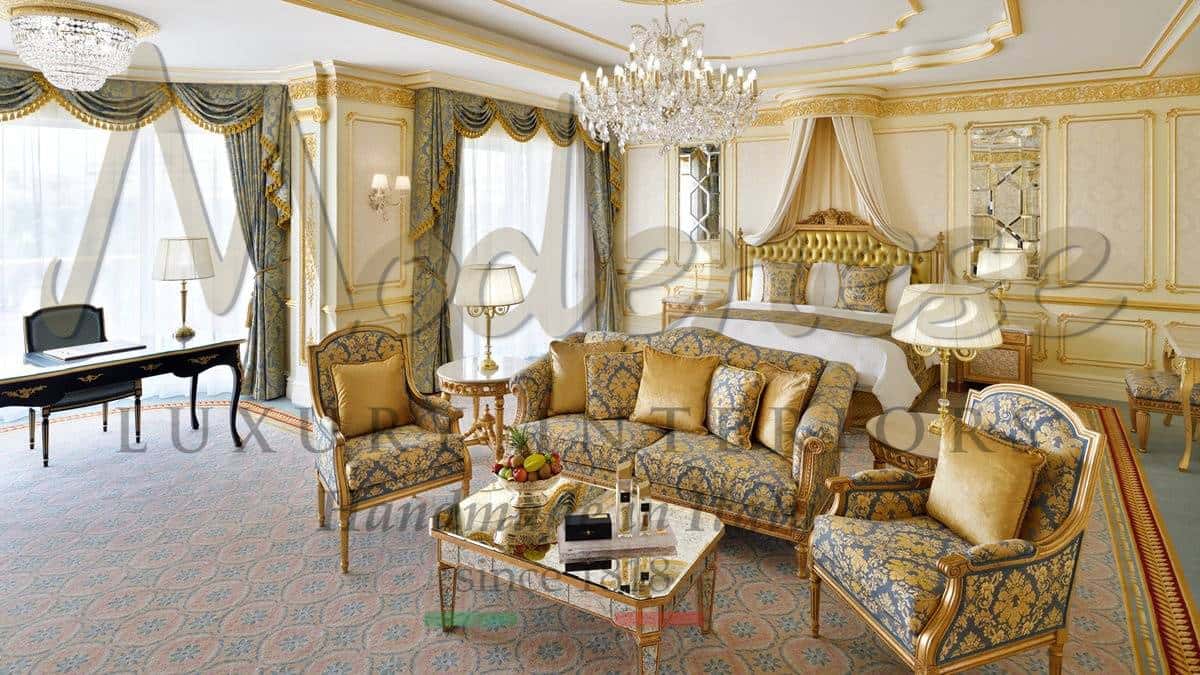The image depicts a lavish and ornate Baroque-style bedroom and sitting room area, with a rich assemblage of intricate details and opulent finishes. The room features handsome wooden paneling and elaborate gold-detailed wallpaper adorning the walls. The carpet boasts a pink and blue floral pattern that complements the overall grandeur of the space. A prominent crystal chandelier hangs from the ceiling, casting light on elegantly upholstered furniture. 

The bed has an exquisite gold-carved headboard, accompanied by wall sconces and mirrors on either side, as well as a round canopy curtain, partially drawn to reveal the meticulous details of the headboard. There are additional golden lamps with embellished bases, and the windows are adorned with grand drapes in hues of blue, green, and gold, enhancing the room's royal aesthetic.

A black and gold desk is positioned to the left, topped with a lamp, and paired with a matching black chair. On the right, a beautiful dark desk stands as a prominent piece of the room’s refined decor. The furniture, including a sofa and chairs, features luxurious golden blue upholstery with gold plant motifs and pillows. The coffee table, placed in front of the sofa, holds a decorative bowl of fruit. The striking golden accents continue on the feet of the chairs, underscoring the room’s opulent theme.

Overall, the image exudes the elegance of a presidential suite, underscored by the sophisticated watermark reading "M-O-D-E-N-E-S-E Modense," faintly visible in the background.